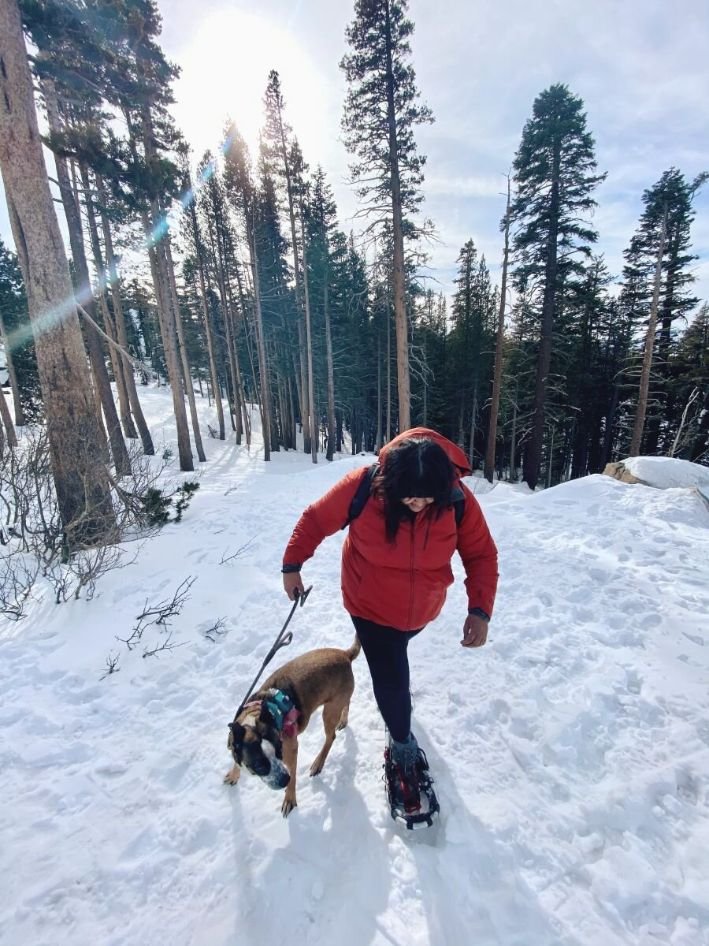In this photo, a woman with long black hair is hiking through a snowy forest, wearing a bright red jacket and black pants. She is equipped with snowshoes to help navigate the thick snow, one snowshoe poised in mid-air behind her, and she carries a backpack. She’s attentively watching where she steps, holding a leash in her right hand that leads to her medium-sized dog, who resembles a bulldog mix. The dog has brown fur with a distinctive white and black-spotted face, and his ears are perked up as he looks forward, also wearing a harness. The backdrop features tall pine and spruce trees, many of which lack lower branches and greenery, offering a stark contrast to the snowy landscape. The sun, positioned behind the pair, casts their shadows toward the viewer, while the sky above is a mix of blue and white with clouds. Beneath their feet, the snow is predominantly white with some patches of light gray interspersed.